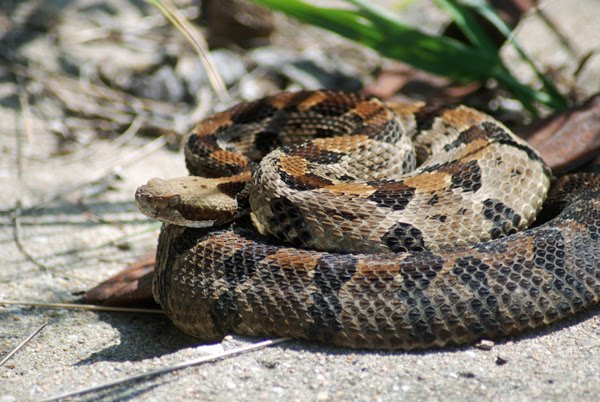The photograph captures a large snake in an outdoor setting, coiled in an intricate spiral on a gray, sandy ground. The snake’s body exhibits a striking pattern of brown and black colors, with some sections featuring dark green and orange hues. Its black spots and lines create a mesmerizing texture that transitions from darker tones at the bottom coil to lighter shades as it ascends, with its head appearing pale in comparison. The snake’s head is oriented towards the left side of the image, giving the impression it might be poised to strike. In the blurred background, there is a plant with green leaves, adding a touch of natural greenery to the otherwise arid scene. The overall photograph is bright and well-lit, clearly taken during the daytime.